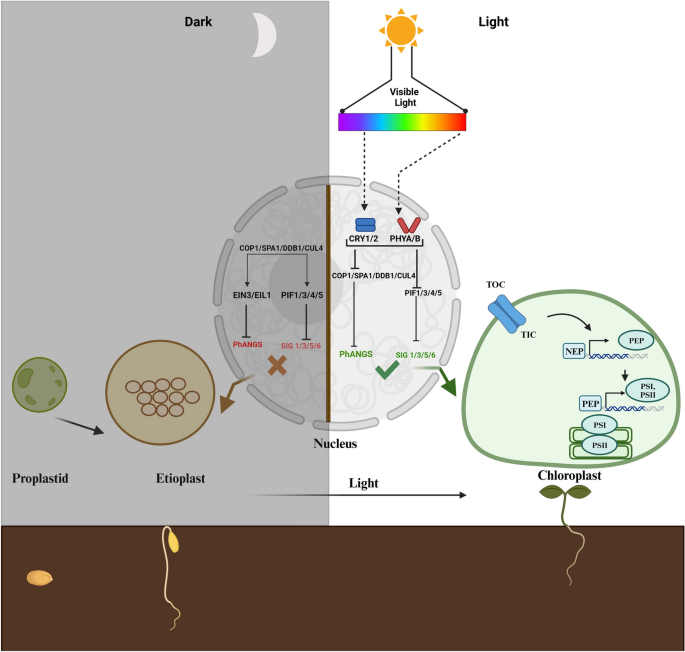The image is a split diagram depicting two contrasting environments: a darker, shadowed left side labeled "dark" with a moon icon, and a lighter, illuminated right side labeled "light" with a sun icon. From the sun, a chart displays the visible light spectrum in rainbow colors (purple, blue, cyan, green, yellow, orange, red) cascading downward. This forms part of a complex flowchart detailing various biological processes.

On the "light" side, arrows point from the sun to several components: two blue rectangles labeled "CRY 1/2," two red V-shaped rectangles labeled "PHY A/B," and further segments including "COP1/SPA1/DDB1/CUL4." There are green arrows leading to "PHANGS" and "STEN 1/3/5/6," with a checkmark indicating these processes. 

On the "dark" side, similar arrows lead to several components indicating different stages of development, with a dashed circle encapsulating terms like "pif 1/3/4/5" and "sig 1/3/5/6."

Additionally, the image contains depictions of plant structures at different stages: a seed on the bottom left under "dark" transitioning to a sprout, and a fully sprouted plant under "light." The presence of terms like "proplastid" with green circles and "chloroplast" associated with sprouted bushes, suggests the biological processes related to plant growth and photosynthesis.